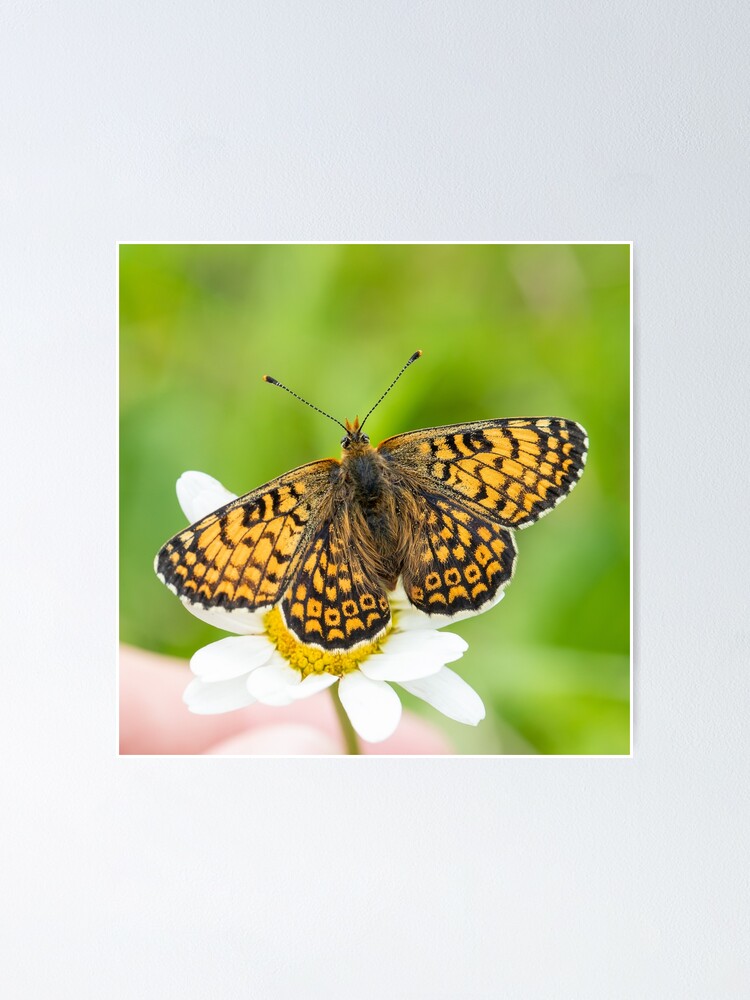This vertically rectangular image is staged and framed with a thick gray border, containing a thin white inner border that surrounds the photograph itself. The photograph was taken outdoors in natural daylight, featuring a softly out-of-focus green vegetation background that appears lighter in the lower left corner and darker in the upper right. Central to the crisp, in-focus area of the image is a delicate white flower with numerous small petals, encircling a vivid yellow center. Perched on this flower is a striking butterfly with its wings fully spread. The wings, primarily a vibrant orange accentuated with black borders and zigzag patterns, display the butterfly’s intricate designs. Its body is mostly black with tufts of yellowish-black hair, and its antennae extend upwards, giving it an elegant poise. Just below this captivating scene, slightly blurred, is the hand of a white person, with their thumb and index finger delicately holding the green stem of the flower, anchoring the visual composition and adding an intimate, human element to the image.